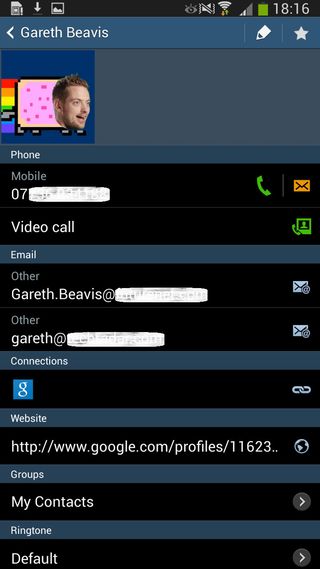Caption: 

"A vibrant and colorful screenshot featuring Gareth Beavis. The image presents Gareth in a spectrum of rainbow colors set against a navy blue background. The interface displays a range of communication options, including ‘Phone’ with a green telephone icon, ‘Video Call’ signified by a picture frame and phone also in green, and 'Email' marked by a yellow icon. Additionally, Gareth’s contact details are shown, including two email addresses and a connection link. The interface also lists various other links and preferences such as his website, Google profiles, groups, my contacts, and ringtone set to default. The alternating black and blue colors further detail the layout, creating a visually striking composition."